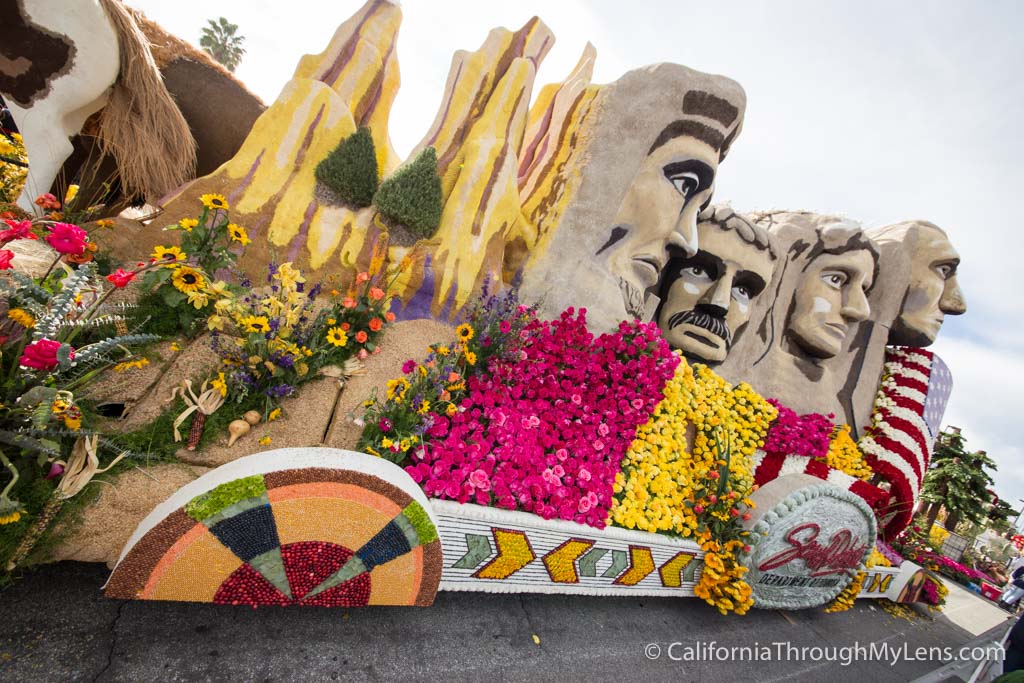The photograph, captured during the day under a bright but overcast sky, depicts a detailed and vibrant Rose Parade float. Central to the float is a striking replica of Mount Rushmore, featuring four meticulously crafted presidential faces set against a predominantly brown mountain backdrop. The float is adorned with an array of floral designs, showcasing an assortment of pink and yellow flowers prominently in the center, and complemented by a red, white, and blue American flag on the right side. Decorative elements include wheels embellished with orange, green, and red glitter. Additional features comprise yellow-topped brown mountains and a creature resembling a cow perched on the float's left top corner. The base of the float is white with directional arrows, accompanied by a gray emblem adorned with red text. Surrounding the float are various other plant decorations. Notably, the image bears a copyright watermark reading "CaliforniaThroughMyLens.com" in the bottom right corner.